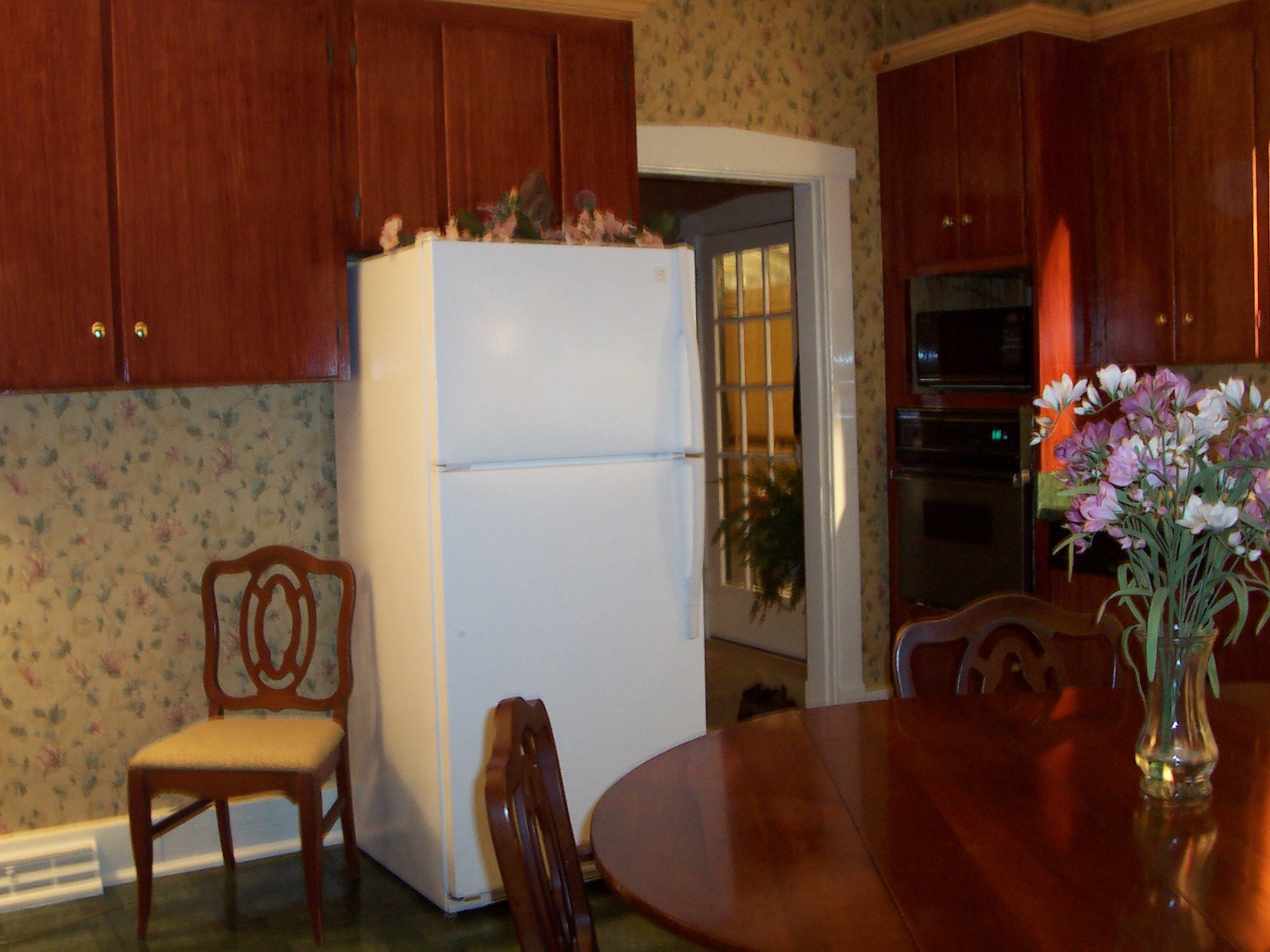The image captures a cozy kitchen and dining area featuring a polished dark wood dining table adorned with a clear glass vase containing white and purple flowers along with a touch of greenery. Surrounding the table are dark wood-backed chairs with distinctive double oval designs and padded yellow seats. A white refrigerator with a freezer on top and additional cabinets above is situated to the center-left of the image. Floral-patterned wallpaper serves as a charming backdrop, enhancing the room’s warmth. The kitchen includes dark wood cabinets that match the table and chairs, a microwave placed above an oven, and a noticeable white-framed doorway leading to another glass door. Other details include a baseboard heater, glossy wooden cabinets with small round door pulls, and a serene window that offers a glimpse into another room. The harmonious blend of dark wood furniture, vibrant floral arrangements, and subtly detailed wallpaper encapsulates a welcoming and lived-in kitchen space.